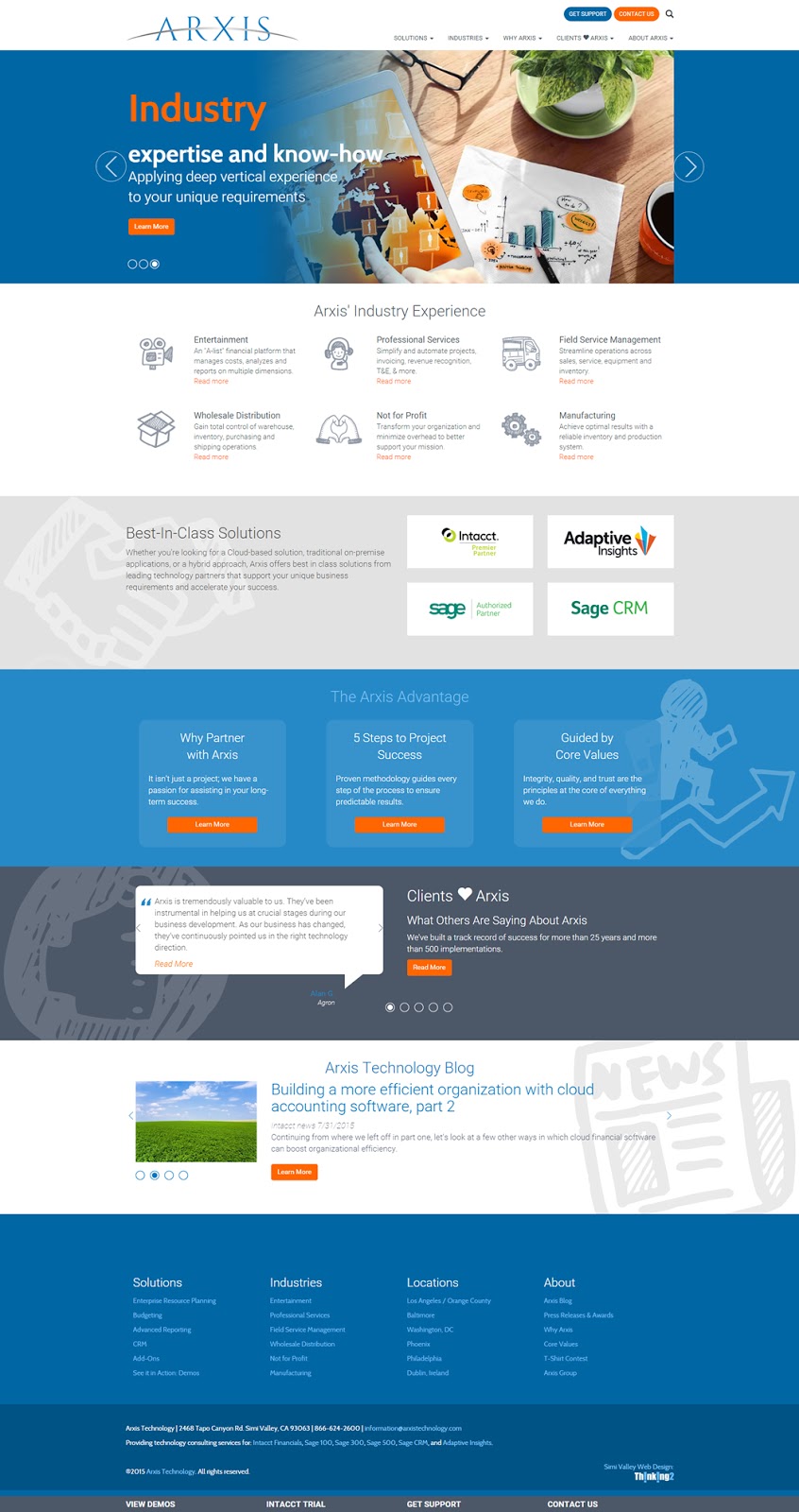This screenshot captures the homepage of ArcSys, a company that's prominently displayed in the top-left corner with its logo. The logo text "ArcSys" (spelled as Alpha, Romeo, X-ray, India, Sierra) is accentuated by a subtle, curved gray line that runs from the initial 'A' to the final 'S', slightly behind the company name. 

To the right of the logo is the main navigation bar with options for "Solutions," "Industries," "Why ArcSys," "Clients," and "About Us." Above this navigation bar are two prominent call-to-action buttons: a blue, pill-shaped "Get Started" button and an orange, pill-shaped "Contact Us" button. Additionally, there is a magnifying glass icon, presumably for a search function.

The central portion of the screenshot features several descriptions about the company's area of expertise, including a header stating, "Industry Expertise and Know-How: Applying Deep Vertical Experience to Your Unique Requirements." Directly beneath this header is a rectangular orange "Learn More" button.

The background imagery includes a varied composition: an eyeglass resting on a table, a green plate with a plant, some abstract illustrations, and a coffee mug. The coffee mug is red with a white interior.

Further down the page, additional descriptions highlight ArcSys' extensive industry experience, detailing their work in Entertainment, Wholesale Distribution, Professional Services, Not-for-Profit sectors, Field Service Management, and Manufacturing.